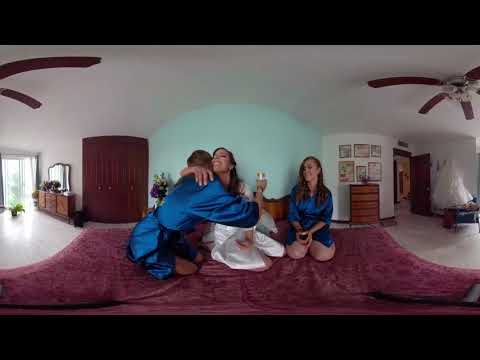In this detailed and slightly distorted fisheye-lens photograph set in a bedroom, three young individuals are sitting on what appears to be a maroon bedspread with a subtle floral pattern. The three are dressed in luxurious, silky bathrobes. On the left, a man draped in a shiny blue velvet robe holds a champagne glass while affectionately hugging a woman in a white silk bathrobe. Another woman, in a matching blue silk robe, is sitting on her knees to the side of the pair, watching them. The setting features notable details such as an overhead ceiling fan with brown blades, a brown dresser partially visible behind the kneeling woman, an open doorway on the right side of the frame, and a sliding glass door to the left. The sliding door allows sunlight to filter in, falling on a plant positioned to catch the rays, highlighting the warm and intimate atmosphere of the room.